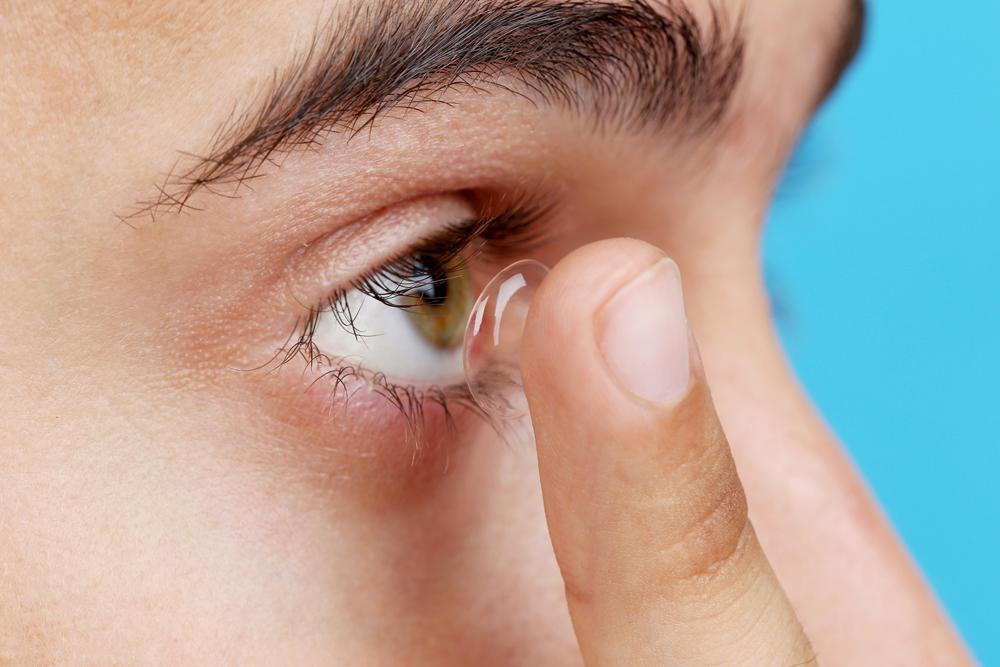This horizontal rectangular close-up photograph captures the intense moment of someone inserting a contact lens into their hazel eye. The image is tightly framed, focusing primarily on the right eye, which is held wide open, emphasizing their readiness to place the contact lens. The person's skin is predominantly clear with a noticeable olive tone, although some redness is visible between the eyebrows. Their dark brown eyelashes are long and curled, with the upper lashes arching upwards and the lower ones curling downwards. The individual's eyebrows are dark brown, slightly unkempt with crisscrossed hairs, and the very beginning of the left eyebrow is also faintly visible.

A finger, presumably the index finger, is poised at the bottom of the frame, less than an inch from the eye, with a transparent contact lens delicately attached to its plain, short fingernail. A segment of the nose's profile appears, along with portions of the brow line, while the background presents a bright turquoise hue, subtly illuminating the scene but keeping the focus sharply on the eye and the contact lens. The detailed skin texture around the eye and the darkened areas around the finger joints add to the intricacy and intimacy of the photograph.